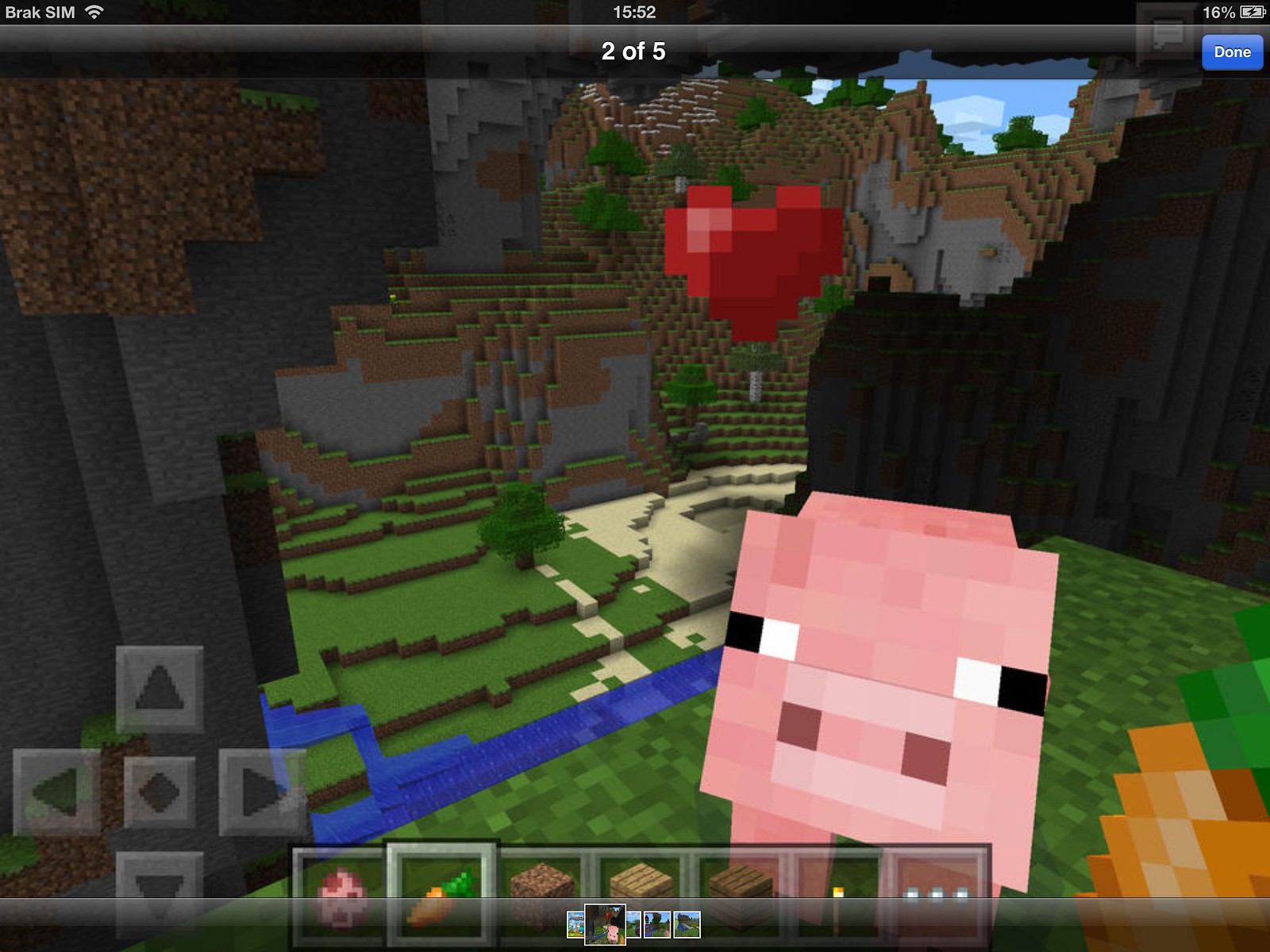Screenshot of the video game Minecraft taken on an old iPhone. The interface shows "BRAX SIM" in the upper left corner with a Wi-Fi symbol, indicating an internet connection. The time is displayed as 1552, with a battery status of 16% at the top right. The image is labeled 2 of 5 with a "done" button in the upper right, suggesting it is part of a photo album. The scene features a pixelated, block-like pig with squared eyes (white and black), a rectangular nose (dark red and pink), and a heart in the middle of the screen. The background depicts a forest surrounded by stone rocks, dirt hills, grass plains, and a beach with water. At the bottom of the screen, there is an inventory bar with various items: an egg with purple dots, a highlighted orange carrot with a green leaf tip, a dirt block, a white wood block, a brown wood block, some torches, and an icon with ellipses.